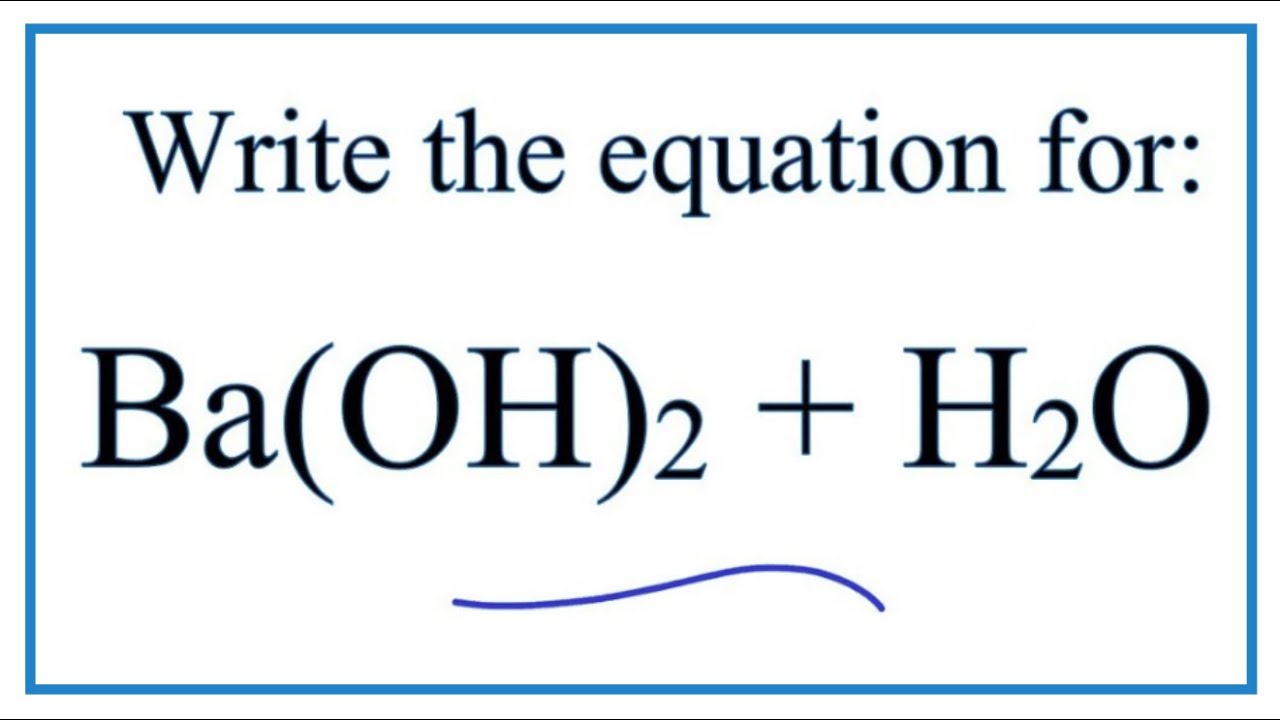The image is a clear, computer-generated graphic depicting a white rectangular card with a thin blue border. Central to the image is a large, bold black text that reads: "Write the equation for BA(OH)₂ + H₂O". This is the chemical equation "BA(OH)₂ + H₂O" prominently presented, with "Write the equation for" written above it in a slightly smaller font. Beneath this text and the chemical equation, there is a wavy or squiggly line drawn in a slightly darker shade of blue. The overall presentation suggests it is part of educational material.